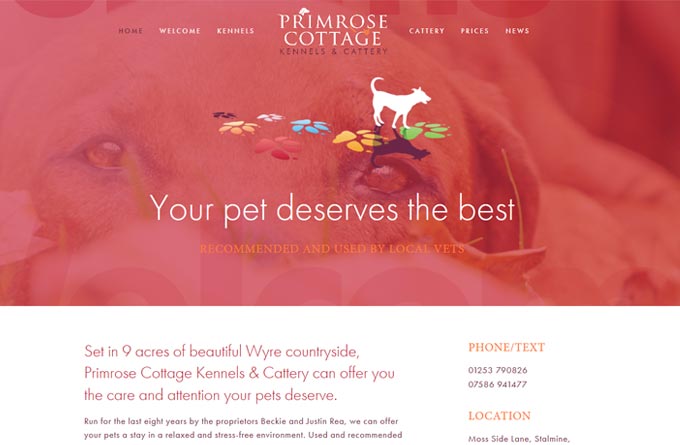The image displays a computer screen featuring a website dedicated to boarding services for cats and dogs. The dominant color on the screen is red, occupying approximately three-quarters from the top towards the bottom. As a background within this red section, there's a close-up, shadowed, and slightly blurred image of a dog, with its eyes being the most discernible feature.

At the top of the website, the navigation menu is displayed with white capital letters. The menu includes items positioned from left to right: "Home," "Welcome," "Kennels," "Primrose Cottage," "Kennels and Cattery," "Cattery," "Prices," and "News." Among these, the words "Primrose Cottage" appear larger, while "Home" and "Kennels and Cattery" are highlighted with a darker font, indicating that "Home" is the current page.

Beneath the navigation, there is a white cartoon outline of a dog, accompanied by brightly colored, large paw prints. Below this image, in a white lowercase font, is the slogan "your pet deserves the best," followed by "RECOMMENDED AND USED BY LOCAL VETS" in orange capital letters.

The bottom section of the website features a white background with text in a maroon or purple font that reads: "Set in nine acres of beautiful Wyre countryside, Primrose Cottage, kennels and cattery can offer you the care and attention your pets deserve." To the right, the contact information is provided with two phone numbers under the labels "phone" and "text," as well as the location "Moss Side Lane, Stalmine."